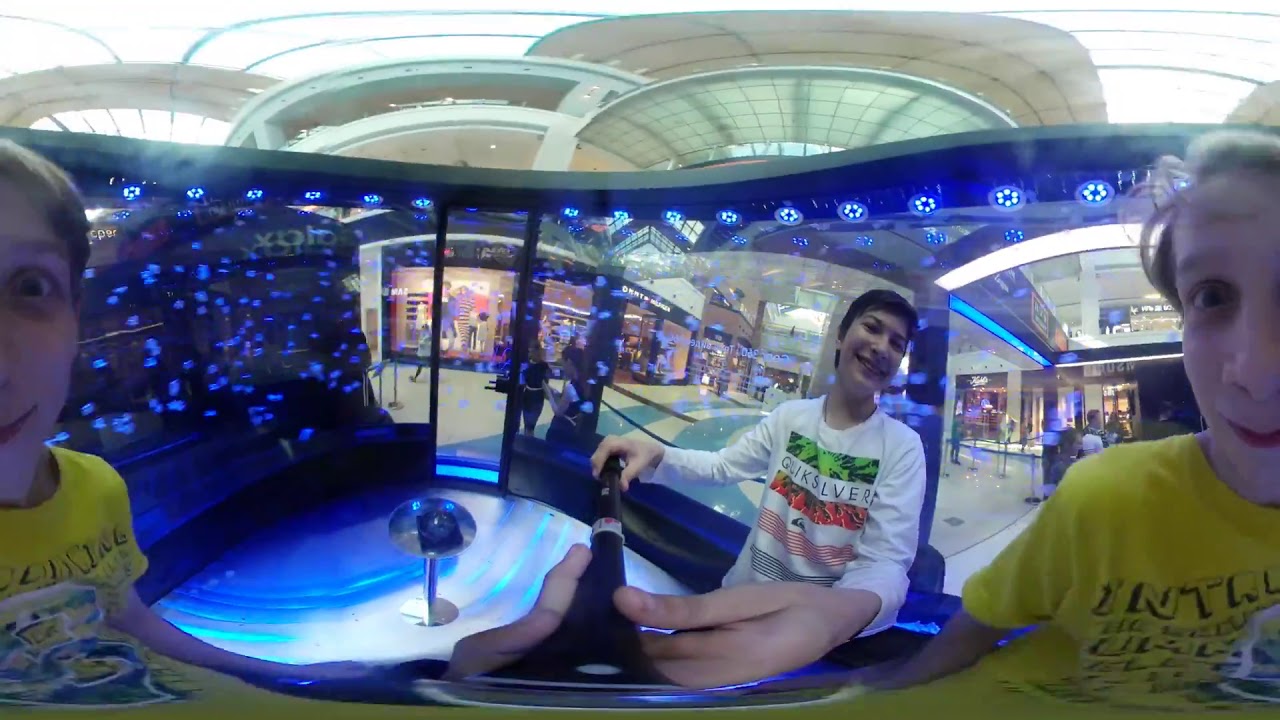The image captures three young individuals in a dark, blue-lit room within a mall, using a GoPro and selfie stick to take a fun and lively photo. The person on the left, wearing a yellow shirt, appears distorted, possibly due to the GoPro's wide-angle lens, creating the impression that both sides of their face are visible at the edges of the image. The individual in the middle, with short-cropped hair and a white, multicolored t-shirt, could be perceived as their parent. On the right, another person in a white shirt is also making amusing expressions. The room features large glass windows and blue lighting that streaks and circles across the walls, contrasting with the shiny floor. In the background, the brightly lit mall area with its light-colored floor and multiple stores is visible, showing several people walking around, adding to the hustle and bustle of the scene. The mall’s design includes round beams emitting light, further enhancing the atmosphere.